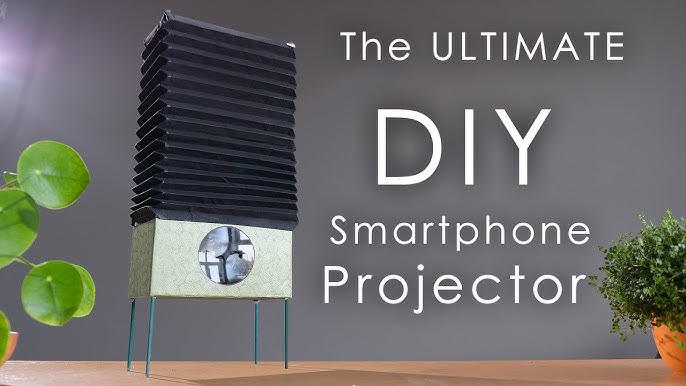The image is an advertisement set against a gray background with prominent white text on the right side that reads "The Ultimate DIY Smartphone Projector." The focal point is a unique smartphone projector on the left, positioned above a tan tabletop. This projector features a white base supported by four slender blue legs and has a distinct accordion-style black top reminiscent of antique cameras. The base of the projector has a large reflective silver or glass circle. The scene is flanked by green foliage: to the left, partially visible circular leaves, and to the right, a terracotta pot housing a fern-like plant, contributing to a clean and simple aesthetic.